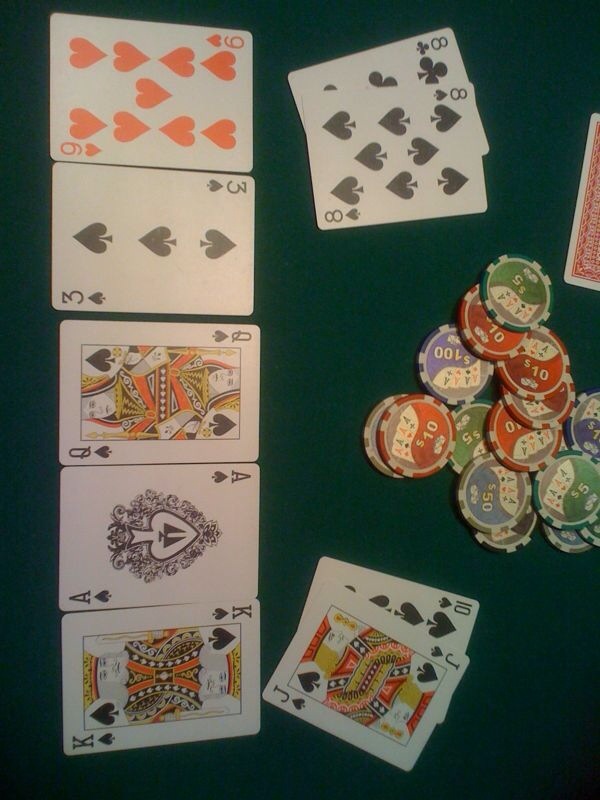This image captures a dynamic scene of a poker game in progress. At the center is a card table adorned with an array of poker chips in distinct denominations. The green chips represent 5, the red chips are worth 10, the blue chips denote 50, and the purple chips are valued at 100.

Arranged on the left side of the table are five face-up playing cards: the nine of hearts, the three of clubs, the queen of diamonds, the ace of spades, and the king of hearts. In the top-right corner of this tableau are two eights, while the bottom-right corner reveals a jack and a ten. Additionally, there is the edge of a face-down card barely visible on the right side of the image, adding an element of mystery to the scene.

The detailed composition of cards and chips sets the stage for an intense game, capturing the suspense and strategic depth of poker.